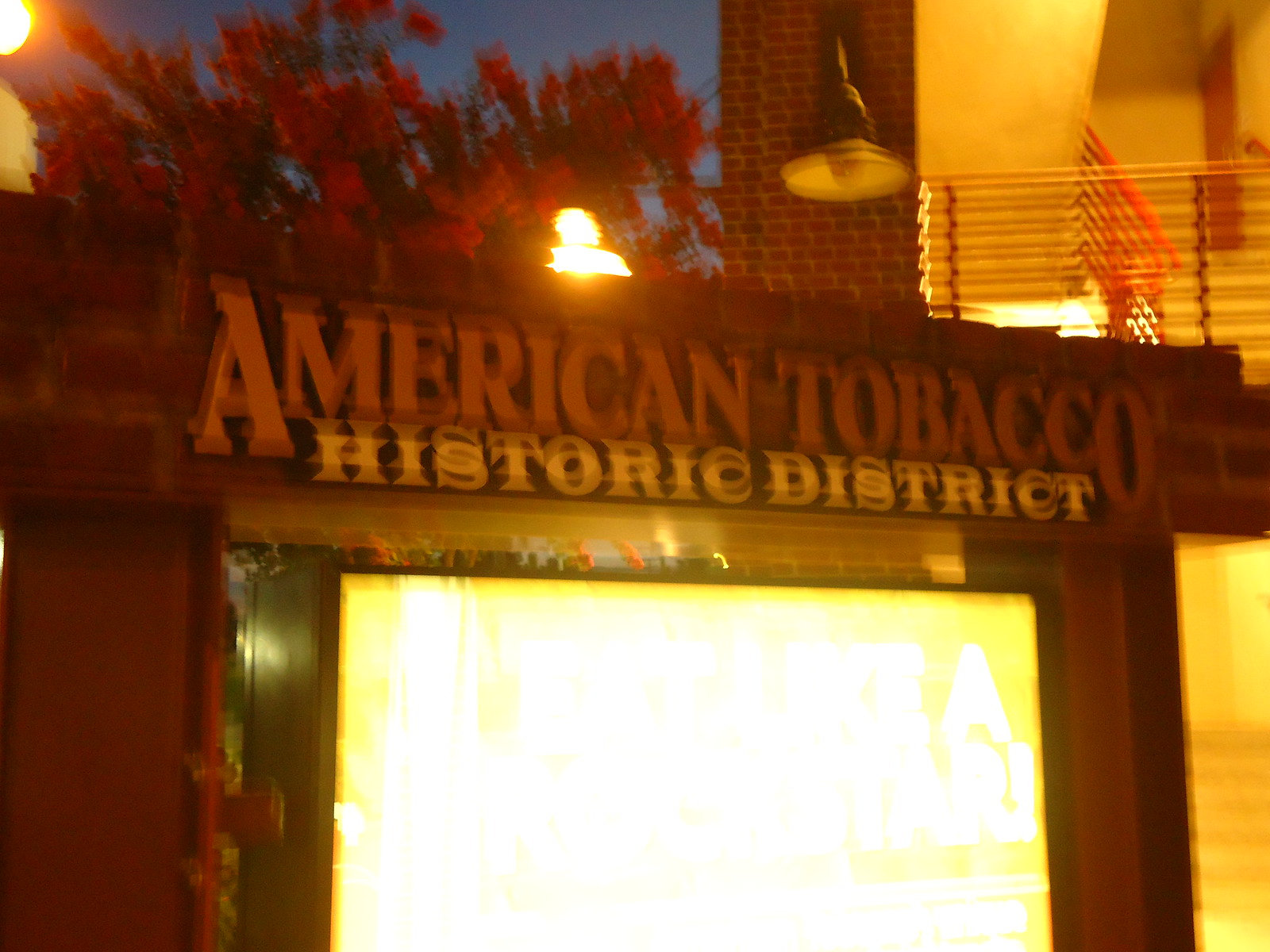This image, taken at night or during the evening, captures the entrance to the American Tobacco Historic District. Dominating the scene is a large sign made of brick that says "American Tobacco" in red letters and "Historic District" in white. Below the sign, an entryway, possibly a door, emits a very bright yellow light, making it difficult to see details inside. To the top left, a tree with reddish leaves and a hanging light are visible, while the top right of the image shows a staircase with a red railing, along with a partially visible red door and white walls. The scene is somewhat blurry, adding a sense of mystery to the historic and brightly lit entryway.